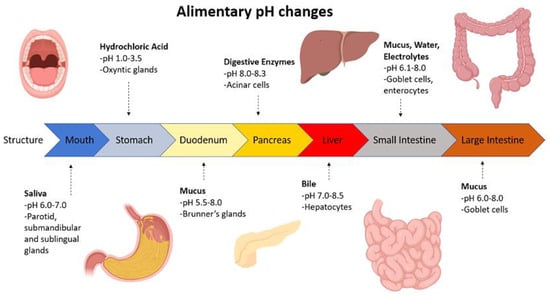This detailed color diagram illustrates the elementary pH changes throughout the human digestive system, segmented by an arrow running vertically down the middle of the image. Starting from the top, the diagram showcases a succession of organs including the mouth, stomach, duodenum, pancreas, liver, small intestine, and large intestine. Each organ is depicted with simple, yet clear illustrations, accompanied by annotations of their respective pH levels and the associated cells or glands responsible.

To the far left, an open mouth is depicted, indicating saliva with a pH range of 6.0 to 7.0, produced by the parotid, submandibular, and sublingual glands. Nearby, an illustration of the stomach highlights the presence of hydrochloric acid with a pH between 1.0 and 3.5, produced by oxyntic glands. Further down, the duodenum is shown, indicating mucus with a wide pH range of 5.5 to 8.0, associated with Brunner's glands.

In the center, there is a drawing of the liver, annotated with bile secretion and a pH of 7.0 to 8.5, produced by hepatocytes. Adjacent to this, the pancreas is represented, showing digestive enzymes with a pH range of 8.0 to 8.3, stemming from acinar cells. The small and large intestines are depicted further along, indicating mucus, water, and electrolytes with pH ranges from 6.1 to 8.0, produced by goblet cells and enterocytes.

The diagram is a comprehensive visual aid, likely designed for educational purposes, that provides a clear overview of how pH levels vary throughout the different stages and organs of the digestive process. For further information, please visit www.FEMA.gov.